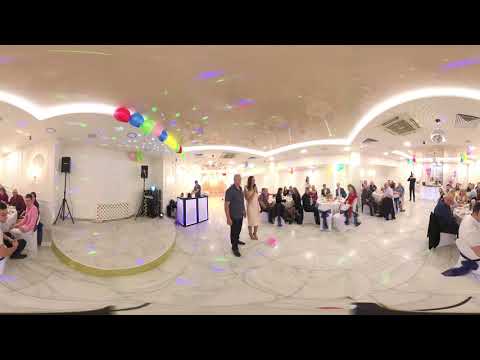A bustling reception takes place in a pristine white room adorned with sleek marble flooring and a softly lit ceiling featuring numerous fluorescent lights. At the center of the image stands a couple, capturing attention: the woman, in a long peach dress, speaks into a microphone, while beside her, a man in a dark short-sleeve button-up shirt, dark pants, and dark shoes accompanies her. Behind them, an illuminated cabinet adds a soft glow to the scene, and colorful balloons in shades of red, green, blue, and yellow hover near the ceiling, enhancing the festive atmosphere. Scattered throughout the room are numerous tables, with guests seated and engaged in conversations, though the details of the tables themselves are indistinct. A small stage with speakers rests against one wall, and a small podium is positioned nearby, contributing to the air of celebration. The room extends to a hallway in the distance, hinting at further activities beyond the frame. Thick black borders on the top and bottom of the image frame the lively scene, encapsulating the celebratory essence of the event.